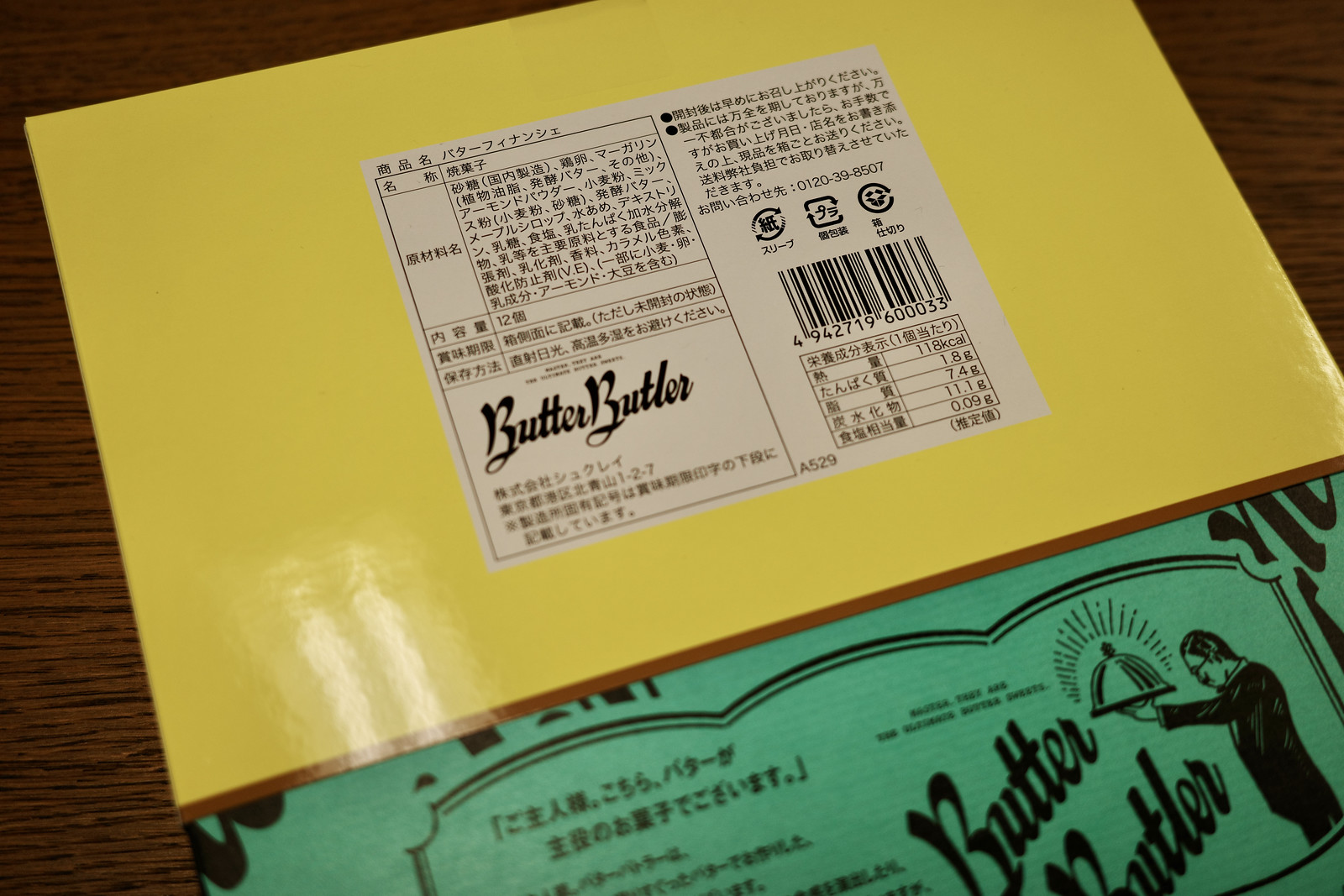The image features two prominently positioned square boxes set against a dark wooden background. The top box is lemon yellow and showcases a white label with abundant dark writing, likely Japanese or Chinese characters. A notable detail in black letters on the bottom left side of the label reads "Butter Butler," along with a visible UPC barcode on the right-hand side. The yellow box also displays nutritional information such as "118 kcal," "1.8g," "7.4g," "11.1g," and "0.09g" next to the barcode. 

Partially visible at the bottom right of the image is the top portion of a green box, also branded with "Butter Butler." Adjacent to this text is an illustrated figure of a butler, dressed formally and holding a dome-covered tray, with more Japanese or Chinese writing on the left side of the green package's label. The overall scene provides a detailed view of the packaging for what appears to be a product marketed under the brand "Butter Butler," featuring both English text and Asian characters.